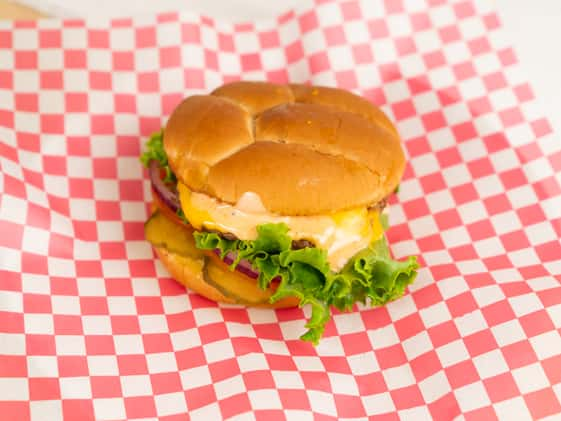A vibrant and colorful cheeseburger is showcased on a red and white checkered deli paper, typical of diner takeout, which is placed on a white surface. The burger features a fluffy, slightly toasted brown bun sliced in two, with the top bun appearing shiny and slightly peach-beige in color. The visually striking ingredients inside include yellow, slightly melting cheese, green lettuce leaves jutting out from the sides, and prominent slices of red tomato and purple onion in the middle. The sides of green pickles are visible at the bottom layer. The checkered paper beneath the burger is slightly creased, accentuating the focus on the fresh, vivid ingredients of the cheeseburger.